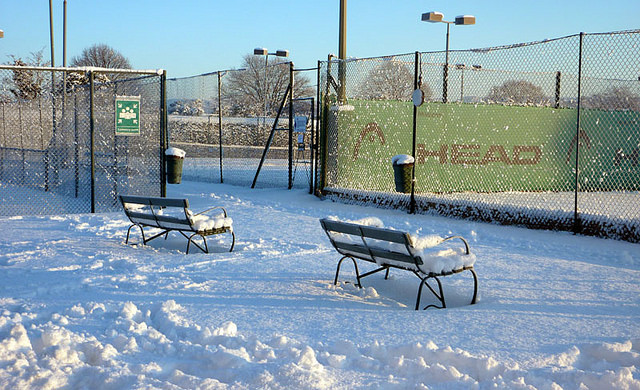A horizontally aligned rectangular image captures a serene winter scene at a sports complex, likely a park or tennis court area, following a snowstorm. In the center of the image are two benches heavily covered in snow, each capable of seating two to three people. The ground beneath and around the benches is also thickly blanketed with snow, and the surrounding area is smooth and undisturbed by footprints.

To the right, a tall wire fence, covered in patches of snow and standing about seven to eight feet high, encloses some of the courts. Attached to this fence are two garbage receptacles, one located more towards the foreground and another to the left. Prominently displayed on a green wall inside the fenced area is the word "HEAD" in big red letters, indicating a brand or sports equipment model. A green and white sign is also visible on the fence, though its message is indistinct from this distance.

Overhead, several light poles with lamps are positioned to illuminate the courts, though they are currently switched off. The photograph is taken under a clear blue sky, adding contrast to the white snow, the green fencing, and the occasional gray fixtures. No people, animals, or vehicles are present, contributing to the tranquil, undisturbed atmosphere of the winter scene.